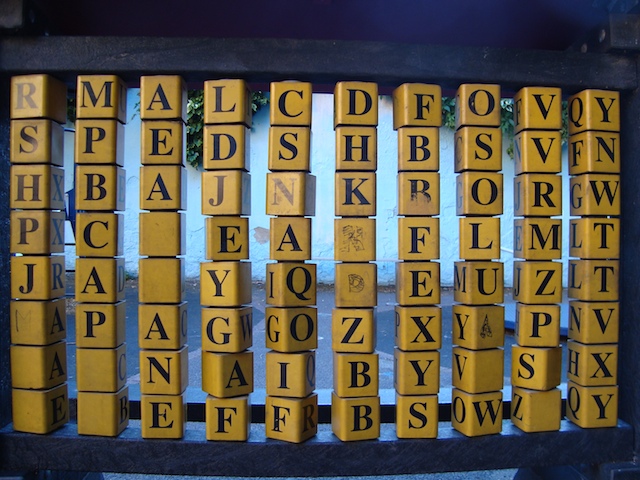This photograph features a children's wooden abacus toy designed not for counting, but for learning letters. The abacus consists of ten rows of wooden blocks, each about an inch high and wide, making them square in shape. These blocks are bright yellow with black lettering, and they're attached such that they can rotate on rods running through their centers. Each block face features letters, with some blocks having handwritten letters on them, as seen in the center right of the image, where an 'R' and a 'D' are added beneath printed 'K' and 'Z'. The blocks seem to have three letters and one blank side. The abacus is fixed within a blue, wooden enclosure. The entire toy is placed by a window, behind which one can see an alleyway or street with a house or white wall covered partially by overhanging tree branches or shrubs.